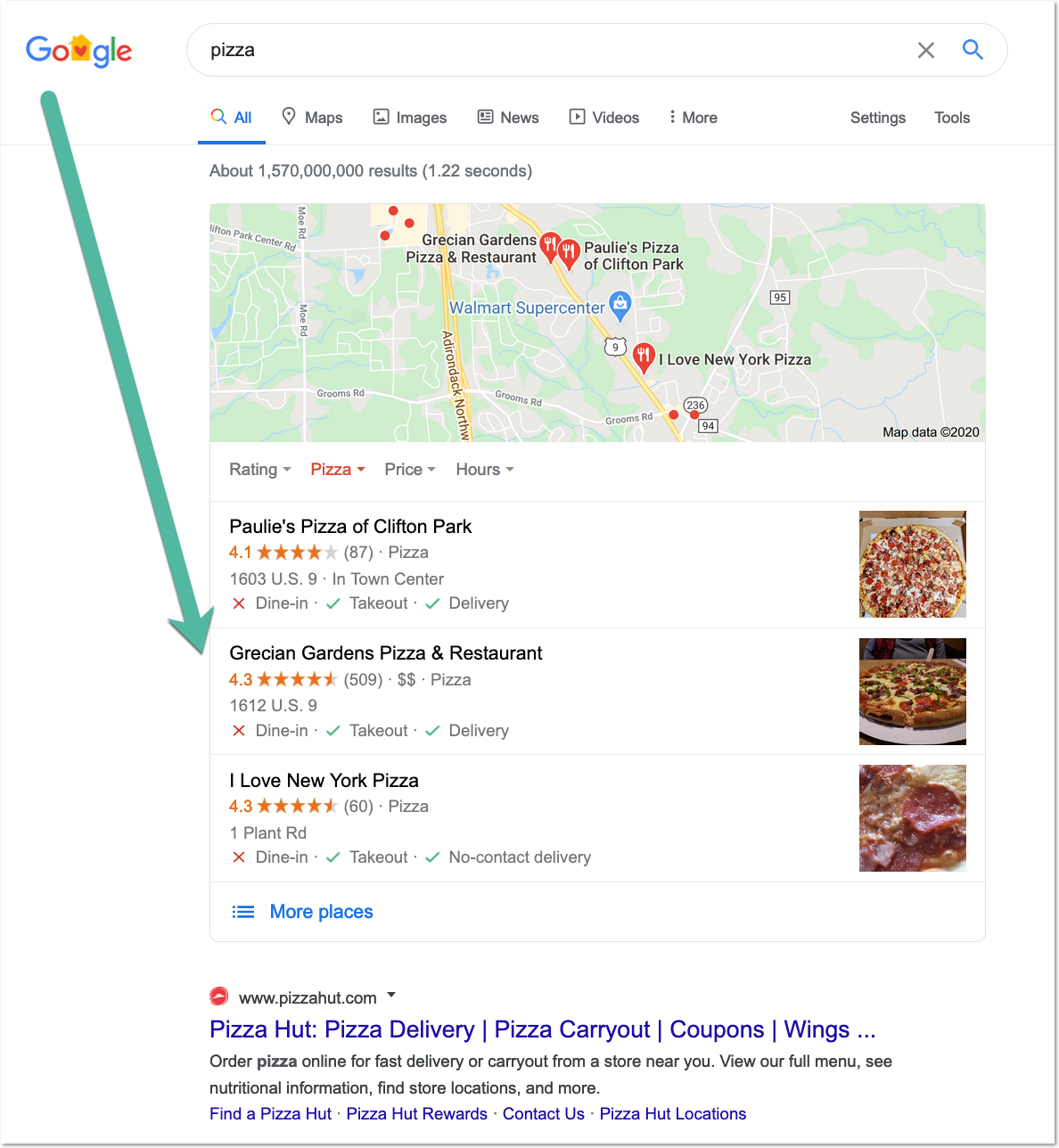A detailed web search result page for "pizza" on Google is vivid with options and information. The results are currently highlighted under the "All" tab, but users can also navigate to "Maps," "Images," "News," "Videos," and more. At the top of the page, various settings and tools are available to customize the search experience. To the right is an "X" button to clear the search field, and to the left of the word "pizza" stands the iconic Google logo, which features a house with a heart symbol inside.

Just beneath the "All" button, the search result statistics are displayed prominently: approximately 1,570,000 results were found in 1.22 seconds. Below this, a map is included, pinpointing various eateries with red markers, and an overlay of a fork and knife symbol indicating food locations. Featured establishments include Gratian's Garden Pizza and Restaurant, Polly's Pizza of Clifton, and a Walmart Supercenter marked in blue with a shopping bag icon. Another notable pizzeria is I Love New York Pizza. The map illustrates different routes in yellow, with smaller streets shown in white.

Further down, drop-down boxes for ratings, pizza types, prices, and operational hours provide additional filters. Three specific pizzerias are detailed, displaying names, number of reviews, exact locations, and services offered. For instance, Polly's Pizza includes a picture of their offerings, and indicates takeout and delivery options. Additionally, a section offers more places with varying services. At the bottom, familiar pizza chains like Pizza Hut are also listed, providing additional ordering options.